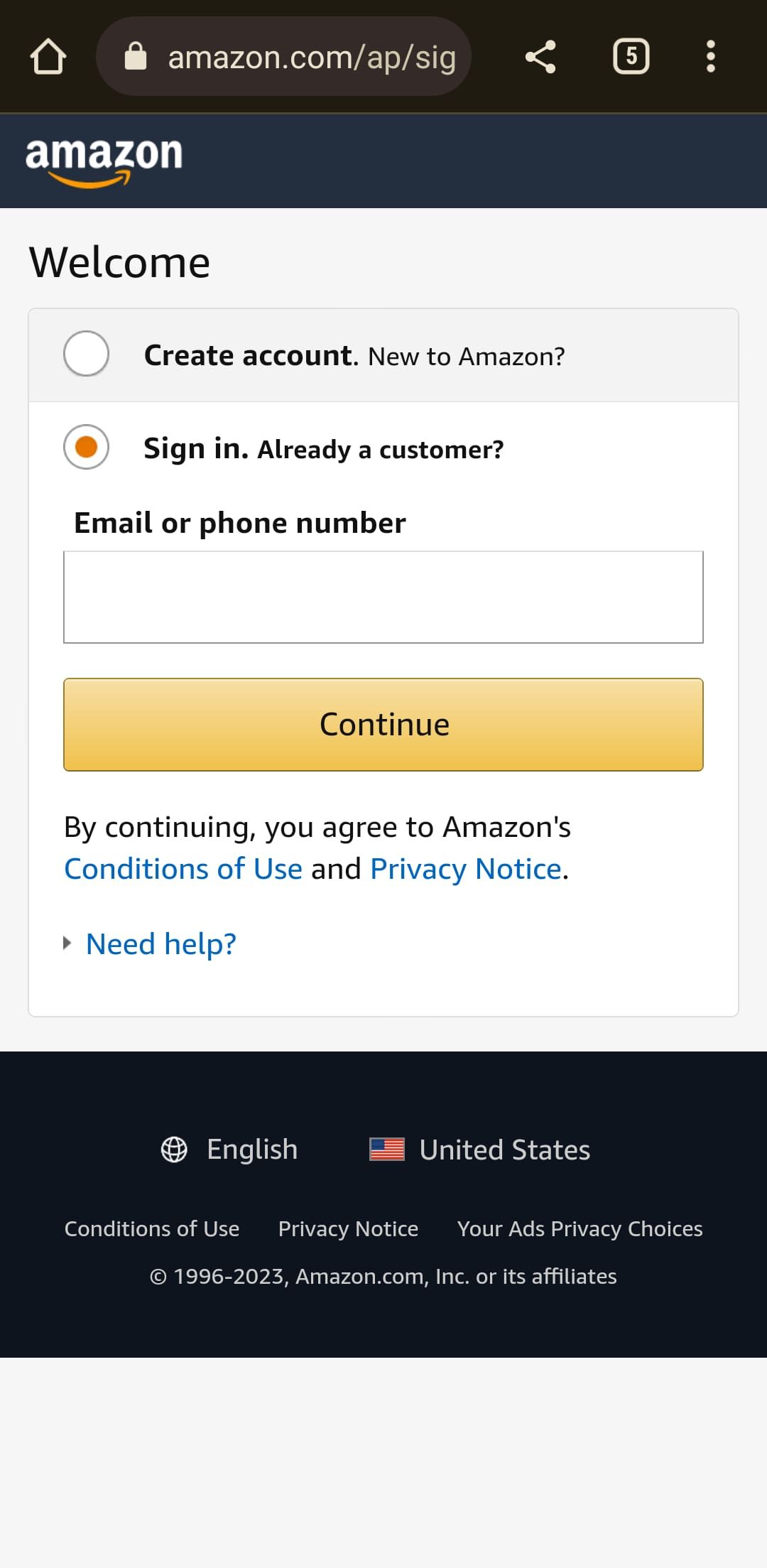The image is a screenshot of an Amazon.com login page. At the top of the page, there is a navigation bar that includes a home icon, a search bar with the address "Amazon.com/app/ap/sig," a share icon, and the number five, likely indicating notifications. 

On the upper left, the iconic Amazon logo is prominently displayed. Below the logo, the page greets users with the word "Welcome." There are two boxes for account access: one labeled "Create account: New to Amazon?" and the second labeled "Sign in: Already a customer?" The latter selection is highlighted in orange.

The form for logging in includes an entry field where users can input their email or phone number, which is currently blank. Beneath this field is a yellow button with the word "Continue" printed in black text. Additional instructions note that by continuing, users agree to Amazon’s "Conditions of Use" and "Privacy Notice," both of which are highlighted in blue to indicate they are clickable links. 

Underneath this, there is a link for users who need help, also highlighted in blue. 

At the bottom of the page, there is a solid black bar featuring white text and an American flag icon. From left to right, the text reads "English," next to the American flag, followed by "United States." Below that are links to "Conditions of Use," "Privacy Notice," and "Your Ads Privacy Choices."

Lastly, the page includes a footer stating, "© 1996-2023, Amazon.com, Inc. or its affiliates."